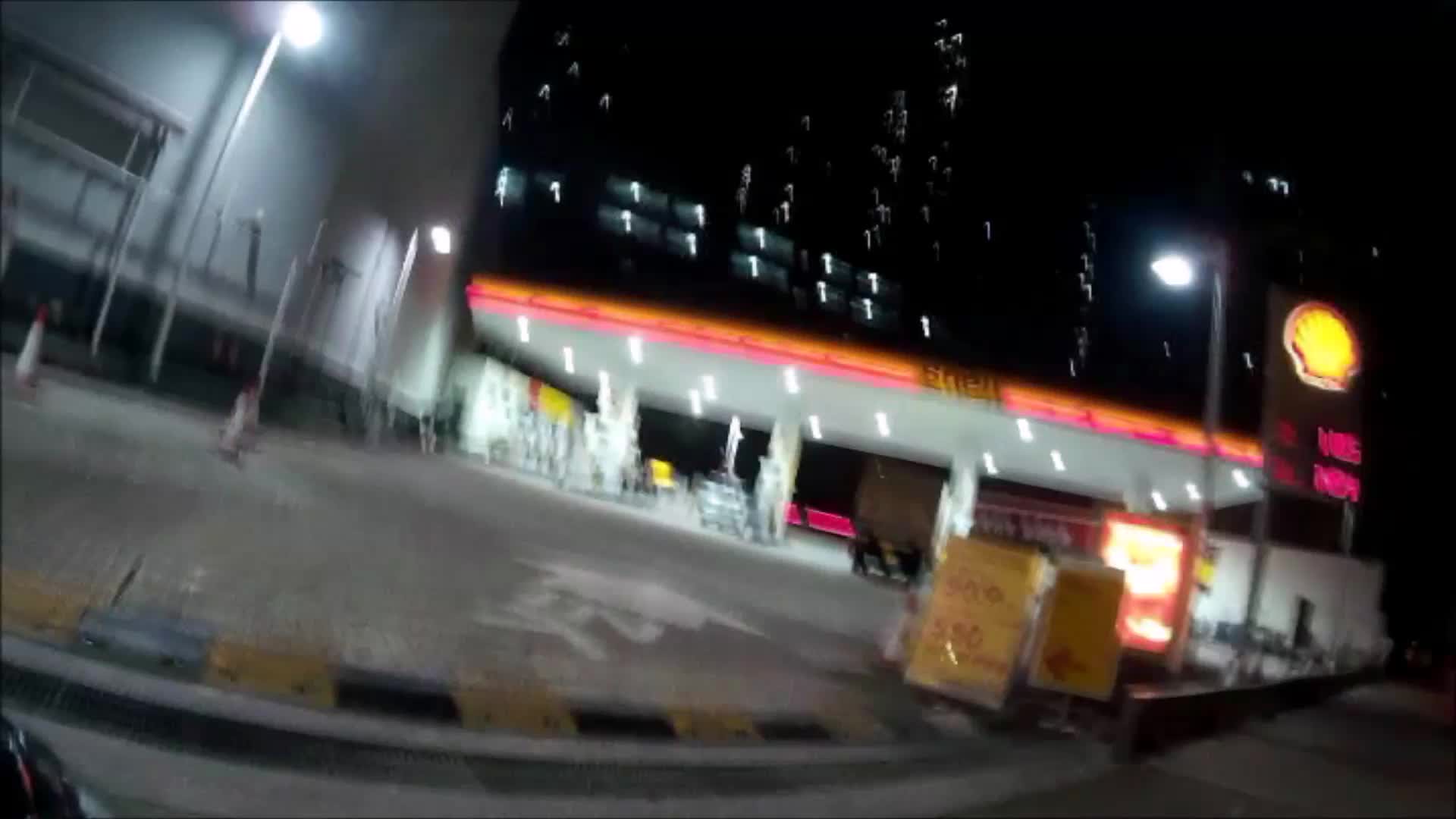This image captures a nighttime scene at a Shell gas station, enveloped in a contrast of darkness and bright artificial light. The station itself is illuminated by vibrant pink and orange accents along the white roof's border, showcasing the Shell emblem in black. There are three gas stalls, one occupied by a black vehicle. To the left, a small, white rectangular store adorned with yellow and red signs stands bright, while in the front, another set of yellow signs with red numbers display blurry fuel prices.

A prominent Shell sign with glowing digital red numbers is visible on the right. Nearby, an array of streetlights with white circular bulbs subtly light up the scene. Adjacent to the gas station, on the left, stands a large white-gray building. The background features the shimmering lights of high-rise buildings, their windows forming a glittering mosaic against the dark night sky. The image captures a mix of concrete ground, low yellow and black walls, and directionally marked sidewalks, all blended in a motion blur that leaves many details slightly obfuscated.